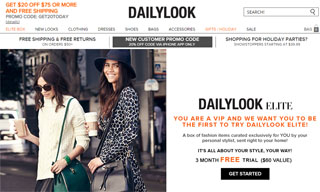This image depicts a webpage from Daily Look, a fashion-related website, possibly a news article, website, or app page, with a slightly blurry text. At the top center, the bold black heading reads "Daily Look," accompanied by a functional search bar on the top right. Prominently displayed on the right side is promotional text for "Daily Look Elite," highlighted in vibrant black, yellow, and orange hues. It reads, "You are a VIP, and we want you to be the first to try Daily Look Elite. It's all about your style, your view. 3 months free trial, $50 value. Get started."

Situated on the top left, the site offers a special deal, "Get $20 off, $75 or more, and free shipping," in attention-grabbing text. Further enticing shoppers, another banner at the top announces "Free shipping and free returns," appealing to holiday party shoppers.

The main visual content features three women dressed stylishly and carrying bags, walking to the left. The woman on the far right dons a black and white coat, paired with a grey handbag and a black hat, her brown hair peeking from underneath. Next to her, the woman in the middle wears a white t-shirt, accessorized with a green bag, a matching green bracelet, a black dress, and black sunglasses, carrying a plastic cup filled with brown coffee. The woman on the far left is also holding a cup, which is white and brown. Both cups appear to be takeaway coffee cups.

Overall, the webpage emphasizes stylish shopping options, exclusive VIP experiences, and promotional deals, tailored for holiday season shopping.